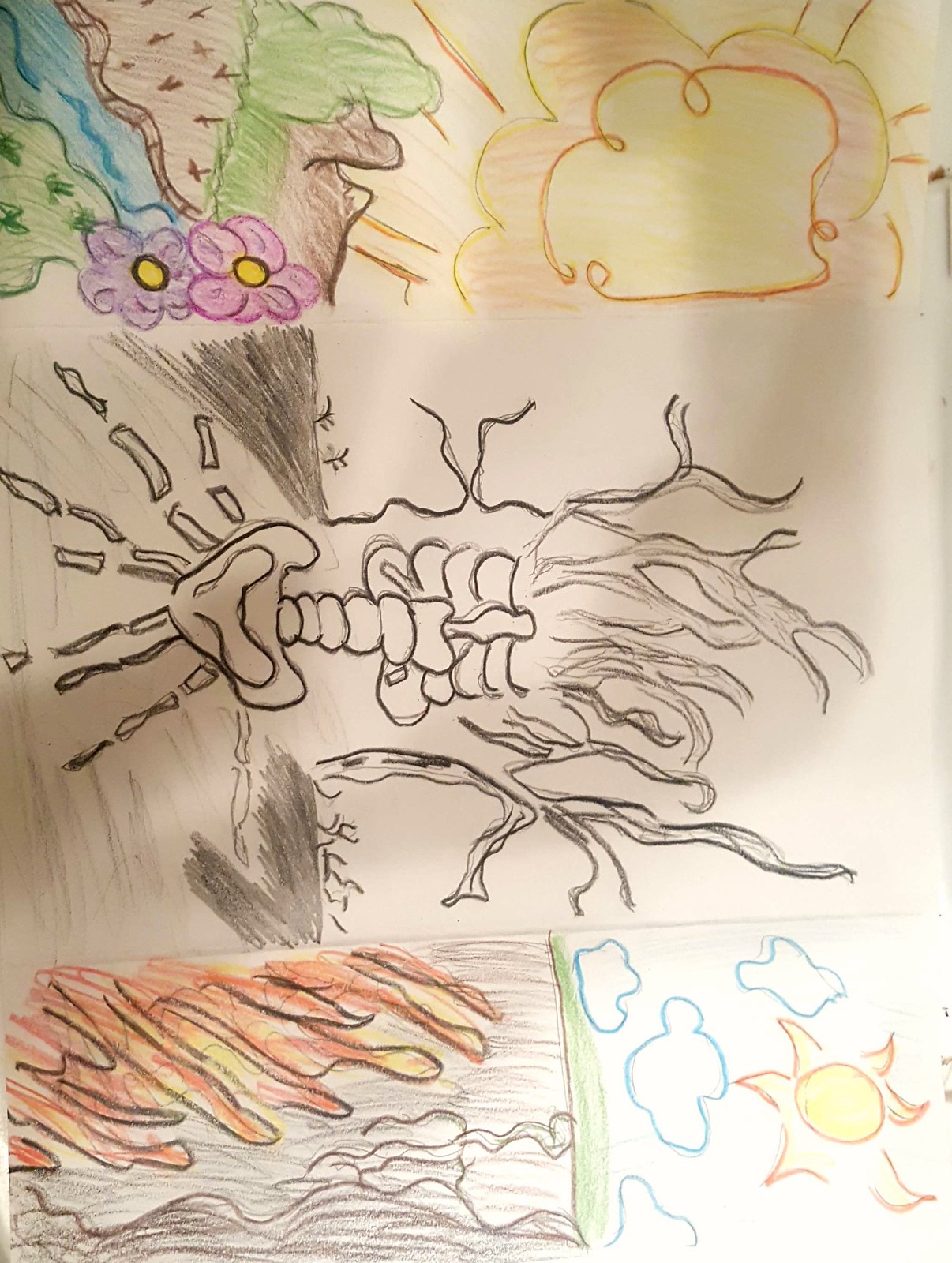A childlike colored pencil drawing, positioned sideways with the top on the right, fills the frame. In the upper right corner stands a simplified sun, surrounded by whimsical clouds. Below, a landscape depicts a scene with flames and a brown sky, conveying an intense, almost apocalyptic feel. On the far right edge of the image, another stylized sun bursts in blotchy brilliance across the sky. Beneath this vibrant sun, a picturesque landscape unfolds, featuring a winding river, stretches of land, and rich greenery dotted with a few charming flowers. Dominating the center of the drawing is an arid, brown road, seemingly desolate, accentuated by skeletal and tree-like shapes, perhaps hinting at a deeper narrative waiting to be discovered.